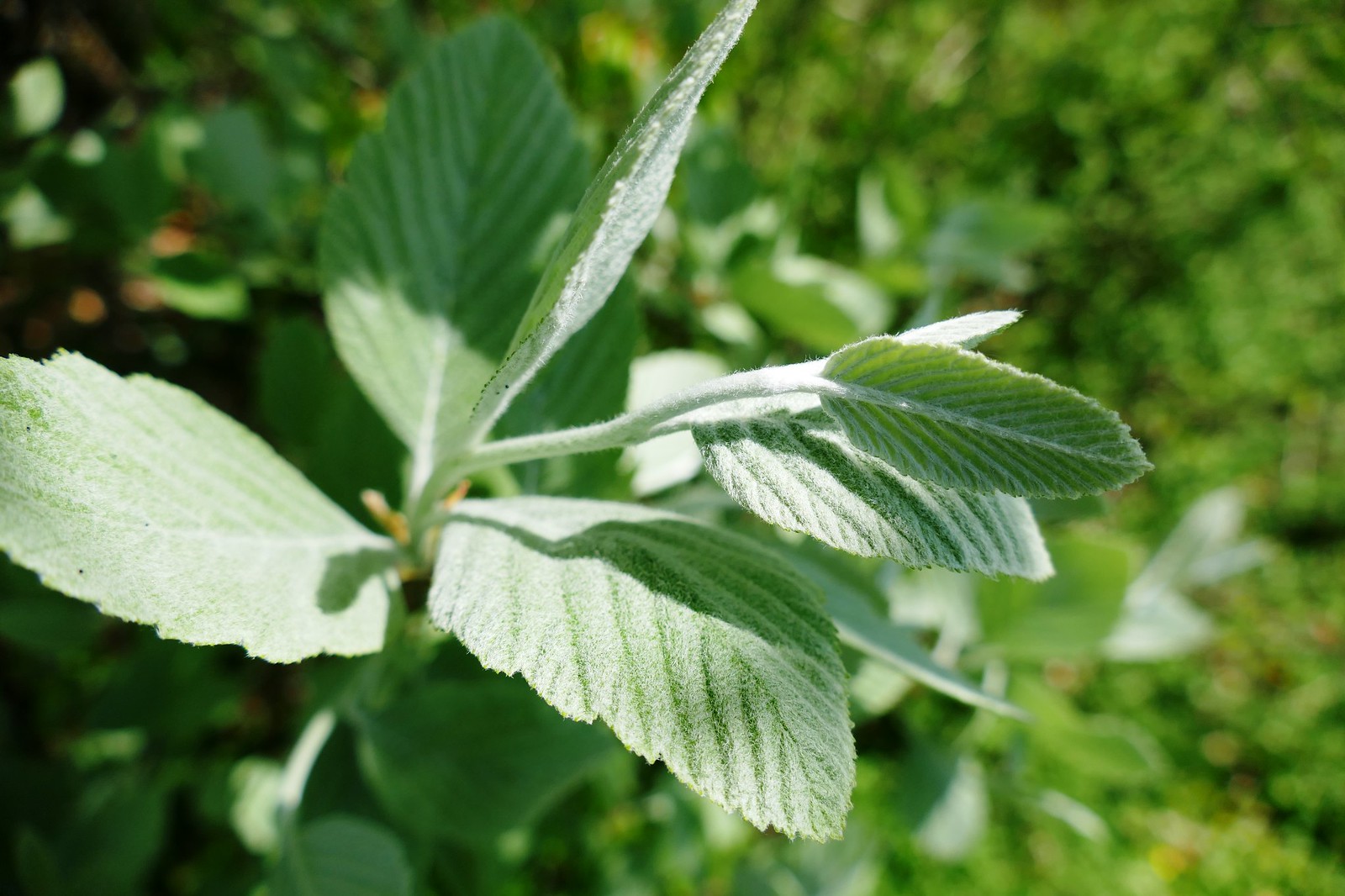The image showcases a close-up of a tall, minty green plant positioned outdoors under bright, sunny conditions. The plant's leaves, which exhibit a velvety or fuzzy texture, feature prominent dark green veins running vertically. These leaves are not entirely smooth and are accentuated by a white frosty appearance, adding to their intricate detail. The plant extends from the left-hand side of the image, reaching upwards and spanning across the frame with several leaves along the central stalk, some large and some tiny. Notably, there are at least eight leaves on the plant, and small yellow bulbs, possibly nascent flowers, are visible further down on the stem. The background of the image is entirely blurred with a bokeh effect, composed of various shades of green, white, and black, creating a mottled yet indistinguishable backdrop. The lighting showcases a contrast with darker regions on the left side and brighter, sunlit areas on the right, reflecting off the surrounding foliage and hinting at grass and other plants. The overall focus proudly highlights the plant's distinctive frosty and textured leaves against the unfocused, dreamy greenery in the background.